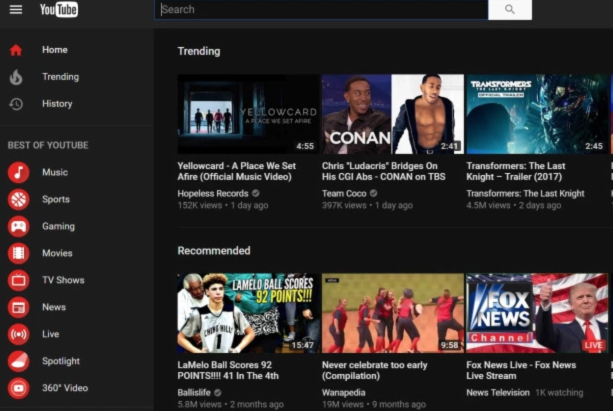**Caption:**

The image captures a YouTube webpage interface, prominently displaying its classic design. At the top-left corner, "YouTube" is distinctly spelled out, adjacent to its logo featuring a tube icon encased within a white background. The site's familiar layout includes a search bar where users can input desired content. On the left sidebar, navigation options, such as "Home," "Trending," and "History," appear. The "Best of YouTube" section follows with categories like "Music," "Sports," "Gaming," "Movies," "TV Shows," "News," "Live," "Spotlight," and "360° Video," each accompanied by a red circle with an icon in the center.

In the main section of the page labeled "Trending," the top video is "Yellowcard - A Place We Set A Fire." Below that, a thumbnail depicts Conan O'Brien on his talk show, showcasing "Chris 'Ludacris' Bridges on His CGI Abs" from "Conan on TBS." Further down is the "Transformers: The Last Knight" trailer, exhibiting a scene from the movie. Following that, LaMelo Ball's impressive feat is highlighted with "LaMelo Ball Scores 92 Points." Another trending video titled "Never Celebrate Too Early" features a girls' baseball team in the middle of a celebratory moment. The list concludes with a "Fox News Live" stream from Fox News.